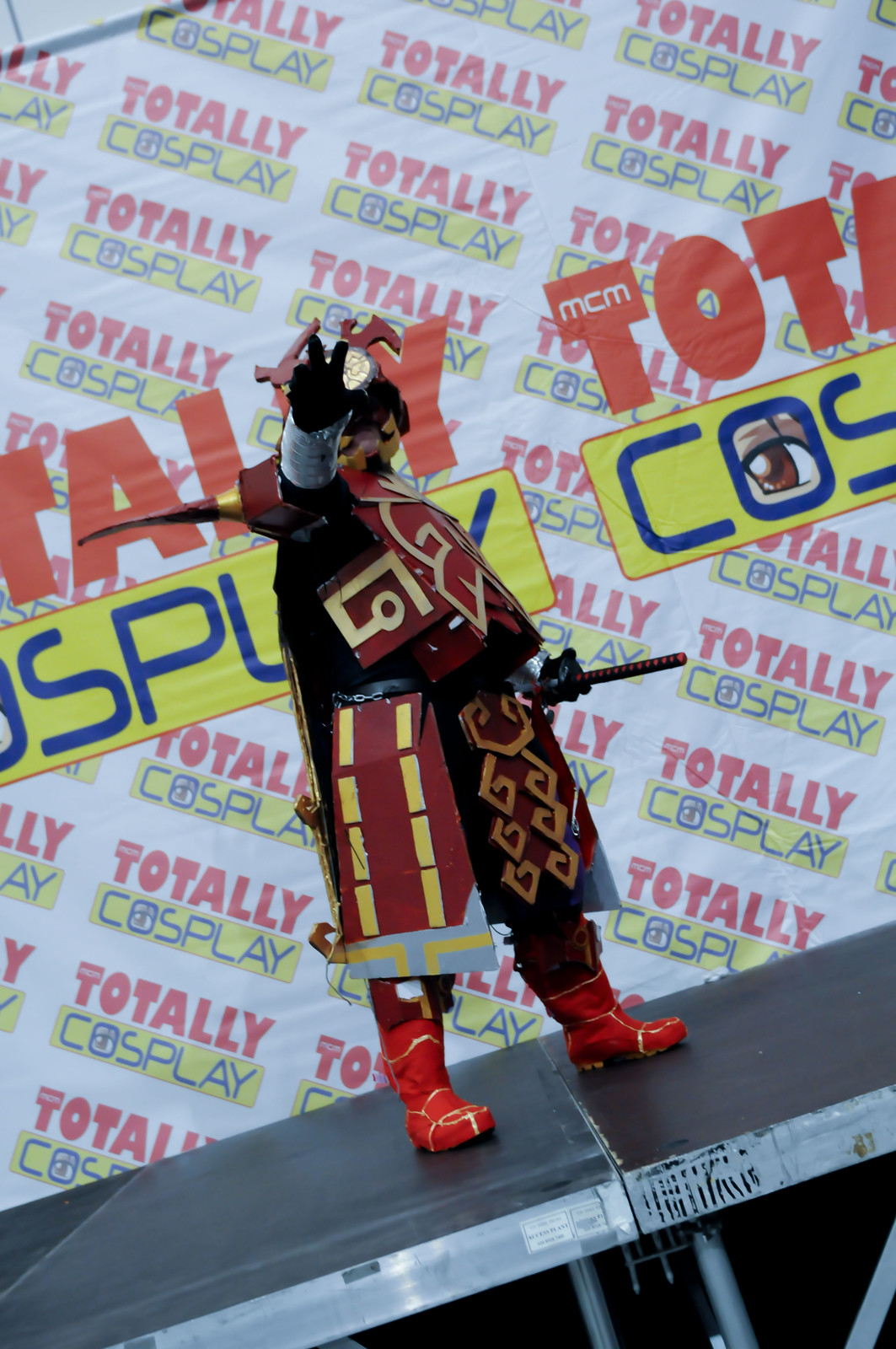This is a vertically aligned rectangular photograph from a cosplay convention, featuring a detailed scene on a black stage. At the center, a person is dressed in an elaborate red and yellow samurai costume, which appears to be crafted from painted cardboard. The costume includes red boots, red and gold armor, and black gloves. The man holds a short sword in his left hand while his right hand is raised towards the audience, perhaps making a sign. His face is partially obscured by a mask with black, closed-eyes design and black hair, and he sports a fake large black mustache. A red helmet partly concealed by his hand completes the attire.

The backdrop is a striking visual, with the words "TOTALLY COSPLAY" repeated diagonally in large, bold letters. "TOTALLY" is in red, and "COSPLAY" in blue, all set against a yellow background. Though the poster's size makes it impossible to view the complete text due to the photograph’s narrow vertical frame, it adds an energetic and thematic touch to the performance scene.